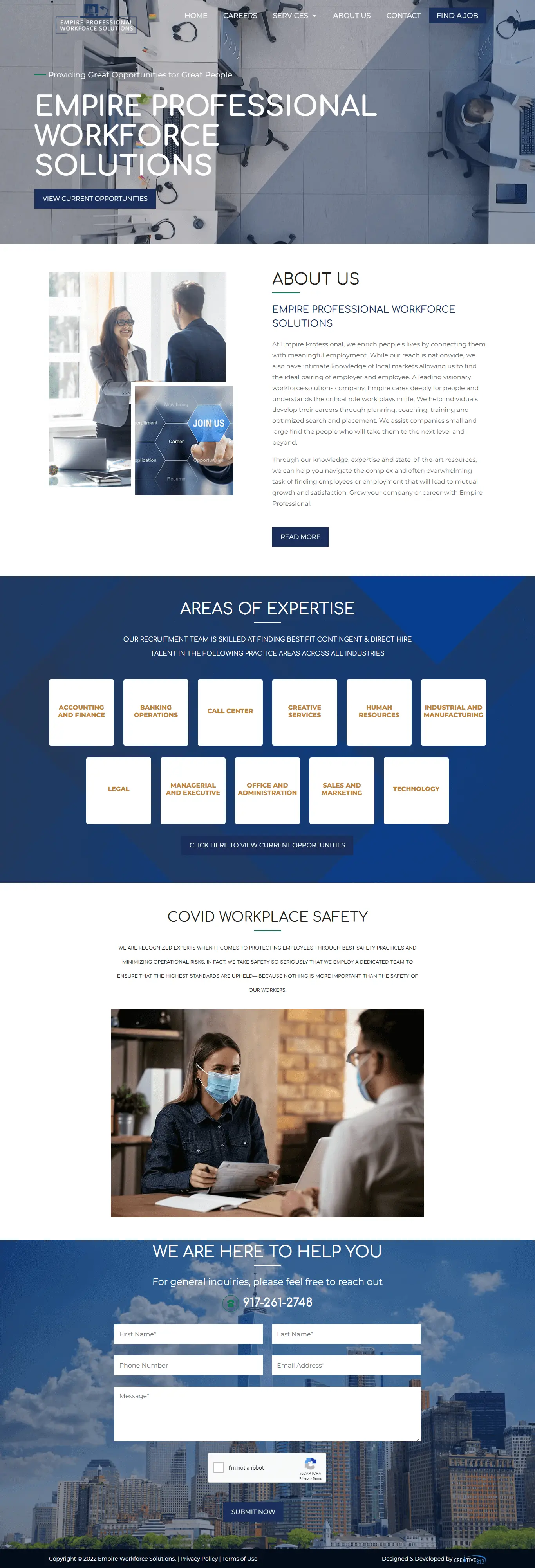The image showcases a website interface for Empire Professional Workforce Solutions, viewed from a zoomed-out perspective. At the top, the website header prominently displays "Empire Professional Workforce Solutions" in white text against a background of an office setting, viewed from a ceiling perspective. This scene includes multiple desks and individuals working.

Below the header, there is an "About Us" section set against a white background. On the left, a photograph portrays two individuals wearing suits, while to the right, there are several paragraphs of small, dense text.

Further down, a section titled "Areas of Expertise" is presented on a blue background. The top row features six white squares with brown text, and beneath them, a second row contains five squares.

Following this, a segment labeled "COVID Workplace Safety" appears, with a brief text description and an image of two people wearing light blue masks in an office environment.

At the bottom of the page, a rectangular image showcases a city skyline with numerous tall buildings. Alongside this image, there is a message stating "We're here to help you" and a form for fielding information that users can fill out.